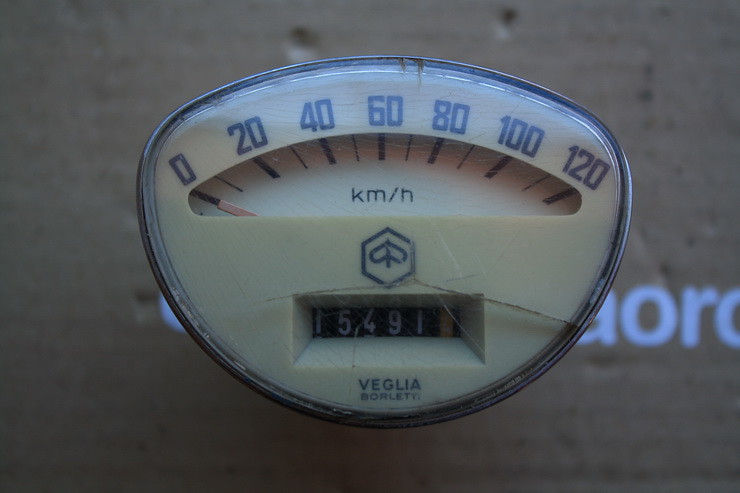A close-up photograph features a vintage meter with a distinct, curvy, diamond-shaped face. The dial is a light cream beige color, elegantly bordered with silver edges. The meter’s face displays numerical intervals marked at 0, 20, 40, 60, 80, 100, and 120, with a prominent dial labeled "KM/8". Beneath the dial, the number "15491" is clearly visible. At the bottom of the meter, the word "BEGLIA" is etched, and in smaller text below it, "BORLETY" is written. The background behind the dial appears to be a textured material resembling cardboard, with partially visible letters "A-O-R-O" extending off to the right. The close-up shot emphasizes the intricate details and craftsmanship of this presumably antique instrument.